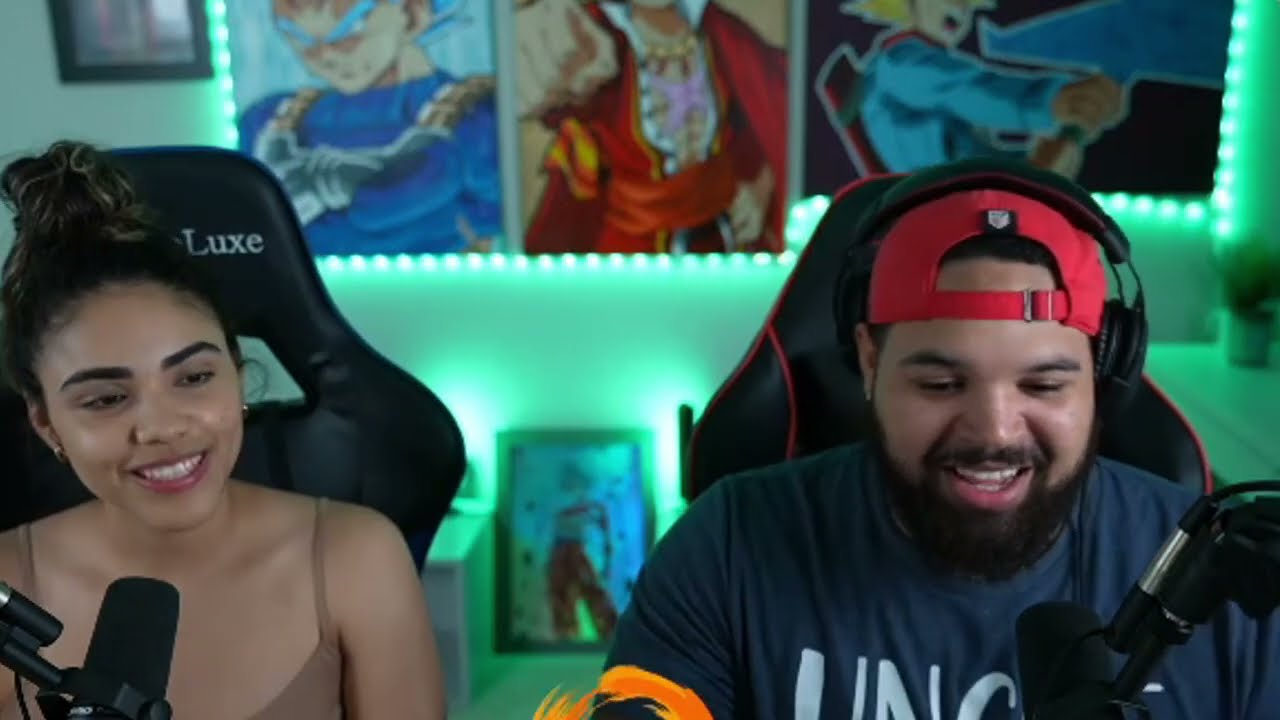In this photograph, two individuals are seated in black, high-backed gaming chairs, facing the camera. On the left side is a young woman with dark hair styled in a bun at the top of her head. She has distinct dark eyebrows, red lipstick, and wears a brown tank top with thin straps, revealing most of her chest and arms. A black microphone extends from the left edge of the image, positioned in front of her. On the right side sits a man with black hair, a beard, and mustache, wearing a red baseball cap backwards. He has dark skin and appears to be speaking or smiling. Dressed in a navy blue t-shirt with white writing, partially visible as "UNC," he also has a microphone extending towards him from the lower right side of the picture. The background features a green wall adorned with three prints, likely depicting characters from the anime Dragon Ball Z, each framed with green neon-type lighting. The setting suggests they might be participating in a radio show or podcast interview.